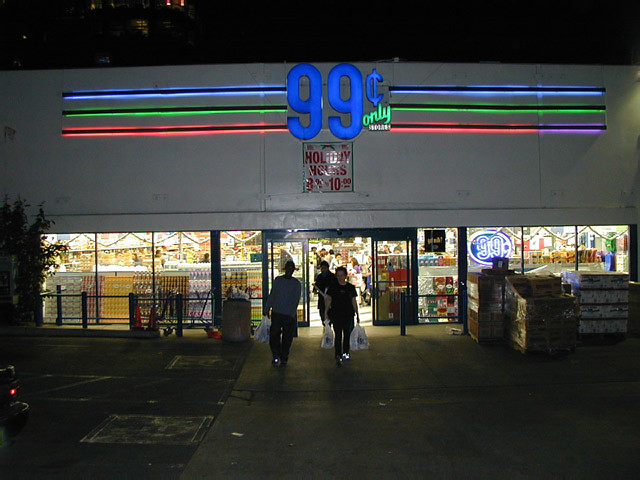The image portrays the vibrant nighttime exterior of a 99-cent only store. Dominating the scene is a prominent neon sign displaying “99¢ ONLY” in large, bright blue digits, with the word “only” in green. Surrounding this is a trio of illuminated stripes—blue, green, and red, with the red stripe showing a purple tint in the middle—running horizontally across the top of the building. Directly beneath the main sign, a white banner with red lettering is partially obscured by glare, though “three for ten dollars” is visible.

In front of the store's entrance, the sliding glass doors are open, revealing glimpses of the well-lit interior crowded with various items. The store also has products displayed outside and in the windows. Three pallets of boxed merchandise wrapped in plastic sit near the entrance, alongside a cart with a trash can.

Several people are seen moving about: one individual is walking into the store, and three others are exiting. Among those exiting, a woman in black yoga pants holds two white bags, a man in a long gray sleeve shirt and dark pants carries another bag, and a second man in a dark blue t-shirt trails behind. In the background to the top right, illuminated windows suggest a tall apartment building.